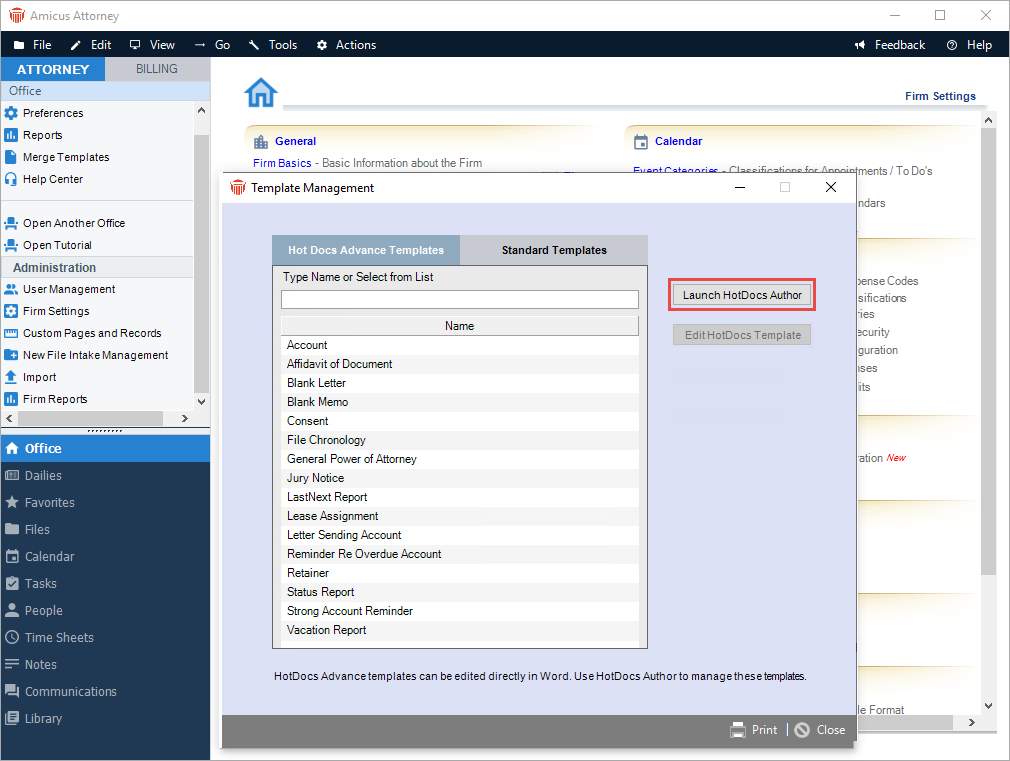A detailed billing form for the attorney, presumably named Armacus or Amacus, is depicted in the image. This main form appears to be issued by the attorney's office after retaining their legal services. The form itself, primarily showcasing the billing information, has sections that are partially obscured by an overlapping window labeled "Template Management." 

The "Template Management" window prompts the user to "type name or select from list" and offers an option to "launch hot docs author." This window lists a variety of document options available for selection, including "account," "affidavit of document," "blank letter," "blank memo," "consent," "general POA," "jury notice," among others.

Despite the overlap, key elements of the main form remain visible. It includes sections such as "references," "reports," and "merge templates." A prominent section, labeled "office," is highlighted in dark blue with a light blue bar displaying its title. Below this bar, several tabs are listed in dark blue text, offering access to "dailies," "favorites," "files," "calendar," "tasks," "people," "time sheets," "notes," "communications," and "library."

The most critical part, the attorney billing section, stands out with a white background and black letters, providing a clear contrast for easy readability. This detailed layout suggests a comprehensive and methodical approach to managing both billing and document templates within the attorney's office system.